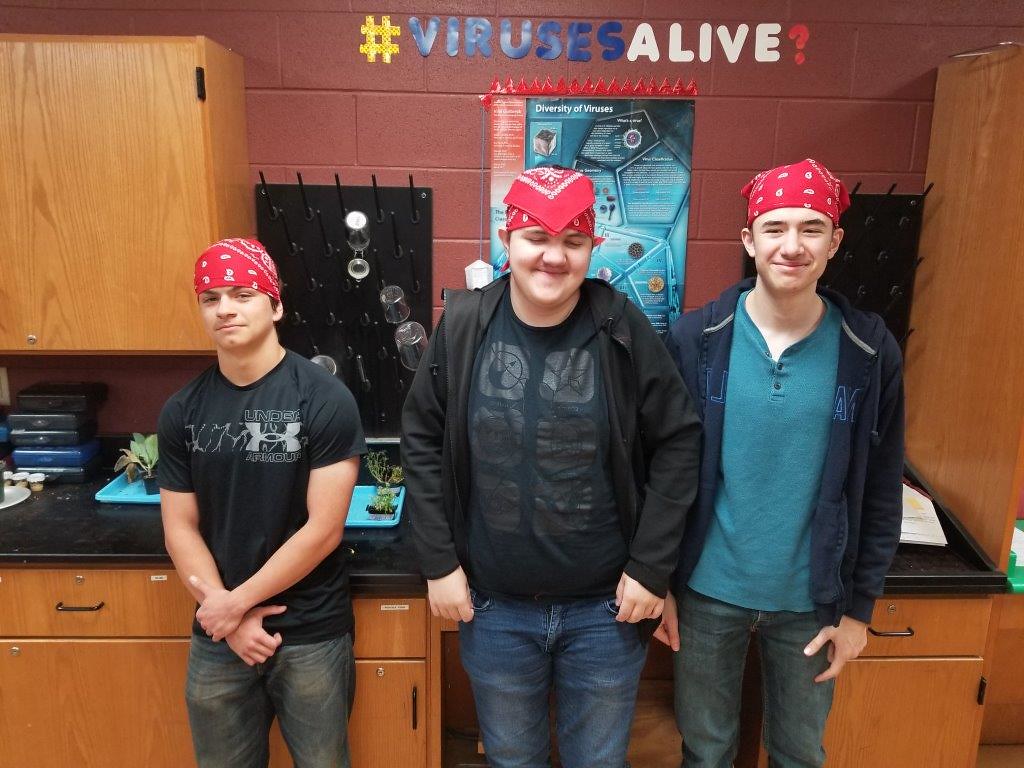In this detailed photograph taken in what appears to be a classroom, three boys stand confidently in front of a wooden cabinet with a black top. Each boy wears a red bandana, reinforcing their coordinated appearance. All three boys are attired in jeans, with the boy on the left dressed in a black t-shirt and folding his arms, his eyes slightly smiling. The boy in the middle sports a black t-shirt under a black hoodie, with his bandana uniquely folded over his forehead, smiling with his eyes closed. The boy on the right, who is also smiling, wears a blue Henley shirt under a hoodie and light black jeans.

Behind them, the backdrop features a vibrant red cinder block wall adorned with cutout letters in yellow, blue, white, and red paper spelling out "#VirusesAlive?" with a question mark. A science poster and various green plants placed on blue trays further decorate the space. The surrounding cabinets are wooden, with black drawer pulls and little gold locks securing the drawers, contributing to the classroom’s organized and studious environment.